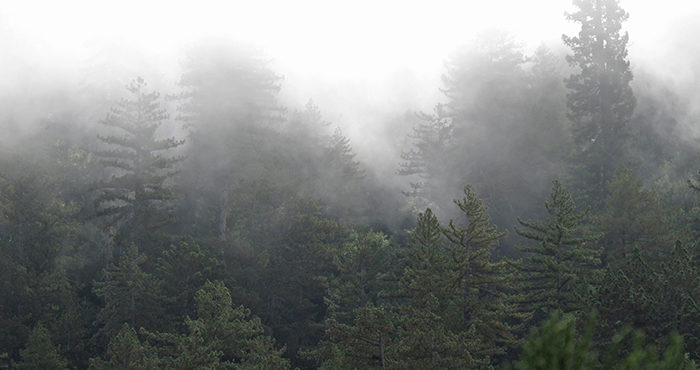This is a daytime outdoor photograph of a dense forest, dominated by tall and healthy green pine trees of varying heights. The image is enveloped in a thick layer of fog, particularly dense towards the left, center, and upper right areas, obscuring the tops of many trees and blending with the overcast white sky. The picture is a close-up, making the greenery of the pine trees at the bottom distinctly visible, while the mid-section shows trees partially veiled by the fog. In the background, the tallest trees punctuate both the left and right sides of the photo, reaching beyond the frame. The mist creates an ethereal ambiance, shrouding the forest in a mystical haze, leaving the ground out of sight and emphasizing the forest's lush, dark green foliage.